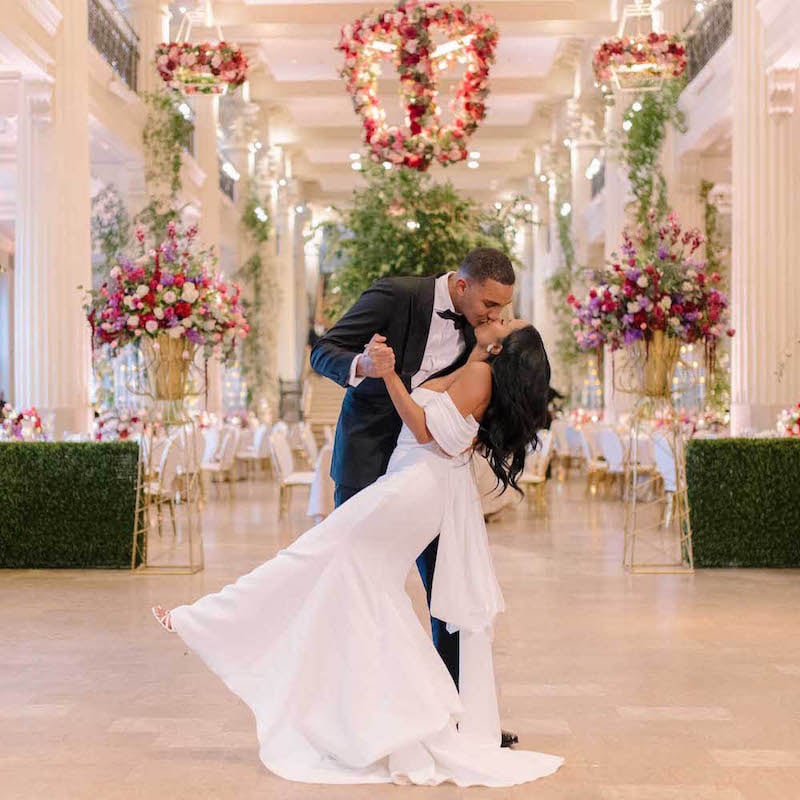In this professionally captured wedding photograph, a groom and his bride are romantically intertwined in a loving kiss. The groom, who has very short, nearly shaven black hair, stands taller than his bride and is elegantly dressed in a black tuxedo with a white shirt and black bow tie. He is holding the bride, dipping her slightly to the right while she raises her left leg and they hold hands, capturing a moment of pure affection. The bride is adorned in a sophisticated white gown that is strapless with off-the-shoulder fabric and features a mermaid silhouette. Her long, wavy black hair cascades down as she leans back, and one can notice her strappy white sandals with her toes peeking out.

They both share light brown skin and are standing on a light beige floor, possibly wood or laminate, which is clear in the foreground. Behind them, the opulent reception hall unfolds, replete with numerous white circular tables and white and gold chairs arranged for guests. The tables are set with floral arrangements, and the ceiling is adorned with garlands of leaves and colorful flowers, showcasing rich hues of pink, purple, red, and white. This luxurious backdrop, featuring large flower pots filled with white, red, and pink blooms amid white columns and soft lighting, accentuates the romantic and celebratory atmosphere of their special moment.